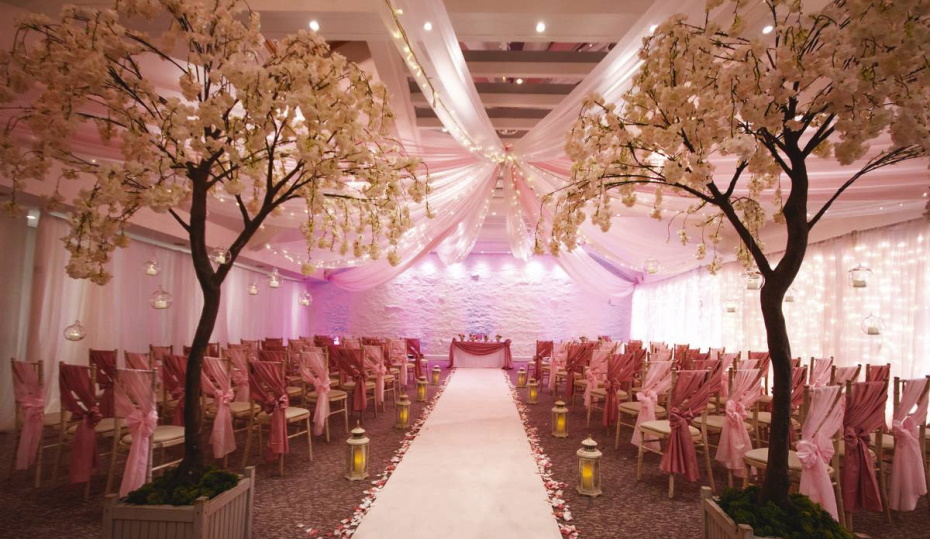This is a landscape-oriented color photograph capturing an elegantly decorated interior room set up for a wedding ceremony. The focal point is a long white aisle carpet adorned with pink and white rose petals and lined with lit lanterns on either side. Rows of chairs, arranged in variably angled groups of three to four, flank the aisle. Each chair is draped in alternating burgundy and pink sashes, tied in large bows that cascade down the left side of the seats.

At the entrance of the aisle stand two cherry blossom trees with white foliage, planted in square white pots with additional green foliage at their bases. These trees anchor the beginning of the aisle leading to the altar, which is dressed with a white cloth and a red tablecloth overlay. Several objects are arranged on the altar, hinting at the ceremony's anticipated rituals.

The ceiling features a star-patterned draping of sheer pink fabric gathered in the center, creating a whimsical yet sophisticated ceiling canopy. The room is infused with a pink lighting effect, enhancing the romantic ambiance. Adding to the ethereal atmosphere are candles in round glass containers, hanging delicately from both sides of the room. The overall style of the photograph is a blend of photographic representationalism and realism, capturing every detailed element with clarity and depth.